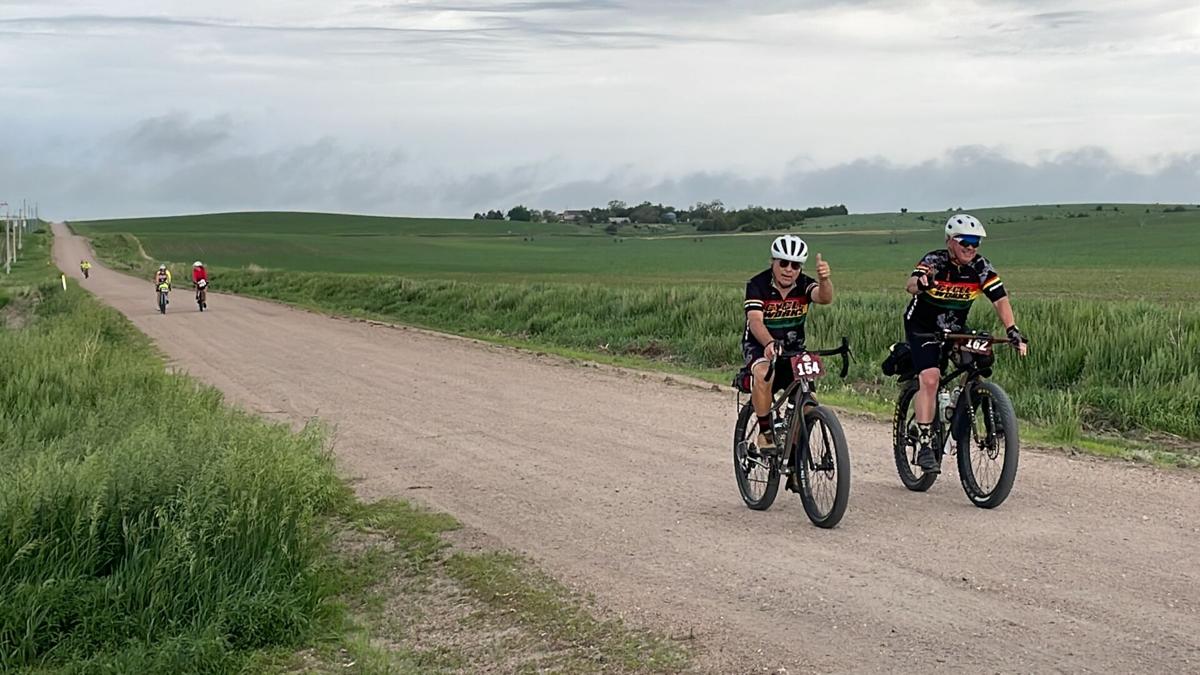This landscape-mode photograph, taken during the day, captures a scene of bikers racing on fat-tired dirt bikes along a rural path. The unpaved dirt road, extending diagonally from the lower left to the middle right of the image, is flanked by tall green grass and patches of wild vegetation. Two cyclists dominate the foreground, both wearing white helmets and black jerseys with orange logos. The cyclist on the left, with bike number 154, is giving a thumbs-up to the camera, while the cyclist next to him, with bike number 162, also has his thumbs up. Behind them, three more bikers can be seen in the distance, continuing along the path that winds through the countryside with rolling hills. The sky overhead is gray and cloudy, creating an overcast, somewhat misty atmosphere. Adding to the rustic charm of this rural scenery are the faint, wispy clouds and a modest fence to the left side of the image.